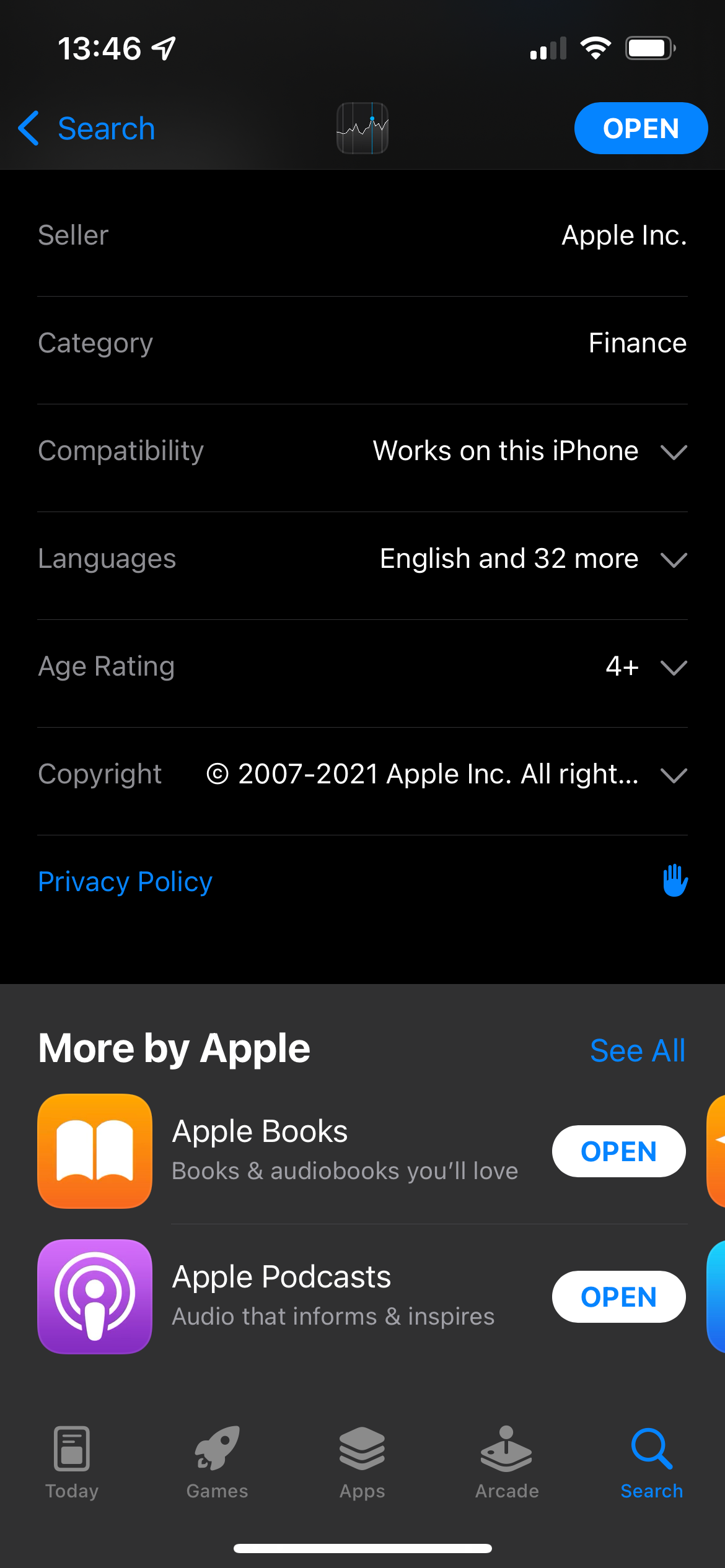The image is a screenshot displaying an app or website interface against a black background. At the top in white text, it reads "1346," accompanied by a paper plane-like airplane icon, a Wi-Fi symbol, and a battery symbol, which is partially blue.

Below these icons, there's a search bar with a back arrow on the left and a small graph icon on the right. Adjacent to it is a blue and white button labeled "Open." Below the search bar, there is a mixture of gray and white text providing details about the app. It states:
- **Seller:** Apple Inc.
- **Category:** Finance
- **Compatibility:** Works on this iPhone (followed by a down arrow)
- **Languages:** English and 32 more (followed by a down arrow)
- **Age Rating:** 4+ (followed by a down arrow)
- **Copyright:** 2007 to 2021 Apple Inc. All rights (cut off text, followed by a down arrow)

Continuing down, a blue hyperlink labeled "Privacy Policy" is accompanied by a small hand icon. Further down, in a gray section, there's a white header "More by Apple" with two app listings:
1. An app with an orange and white open book icon labeled "Apple Books" and a description "Books and audiobooks you'll love" alongside a blue and white "Open" button.
2. An app with a purple icon featuring a person and some rings labeled "Apple Podcasts" and a description "Audio that informs and inspires" alongside another blue and white "Open" button.

Further below, a row of gray icons categorizes different sections:
- **Today:** indicated by a small cell phone icon
- **Games:** marked with a rocket icon
- **Apps:** shown with square icons
- **Arcade:** represented by a joystick icon
- **Search:** depicted with a blue magnifying glass icon

The entire section ends with a white line, demarcating the end of the content.